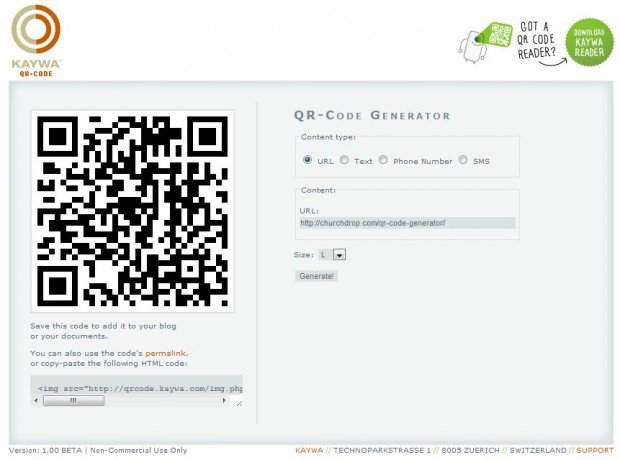This is a detailed screenshot of a QR code generating website, showcasing a smaller, cropped section of the interface. At the top left corner, the KWA logo is prominently displayed, with the text "QR Code" positioned directly beneath it. Adjacent to this, on the right, there is a clipart image of a cell phone with arms and legs. From the phone's camera, a green QR code is being projected. Positioned to the right of this image, the text reads "Got a QR Code Reader?" with an arrow pointing upward toward a green circle that says "Download KWA Reader."

Below the header, a large gray box dominates the space. On the left side of this box is an image of a QR code. Beneath the QR code, the text instructs, "Save this code to add it to your blog or your documents. You can also use the code's permalink or copy-paste the following HTML code." Below this directive is another gray box containing the HTML code with a copy button for easy copying.

On the right side of the large gray box is the QR code generator interface. At the top of this section, the bold text reads "QR Code Generator." Below this, the text "Content Type" is followed by options presented as bubbles for URL, text, phone number, and SMS. Underneath this selection field, a small box labeled "Content" displays the URL to which the QR code will redirect. Further down, the text "Size" appears next to a drop-down box set to "L." Finally, at the bottom of this section, the "Generate" button is prominently featured, allowing users to create their QR code.